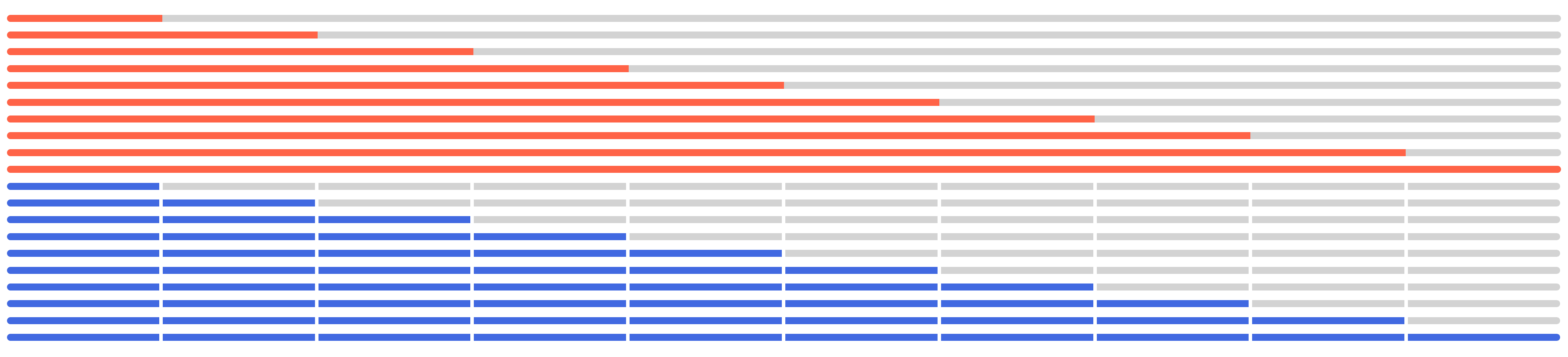The image is a screenshot, likely captured from a computer screen, displaying the top half of the content. The screenshot is of a rectangular area, approximately four to five times wider than it is tall. The background color is white, overlaid with very narrow horizontal gray stripes that run from left to right, suggesting the image is a diagram or a chart of some sort.

In the upper half of the image, there are red horizontal lines that contribute to a jagged pattern. A prominent red line spans the entire width of the image from left to right, while another red line above it extends for a shorter distance, creating a stair-step effect. 

The bottom half of the visible section mirrors this pattern but uses medium blue horizontal lines instead of red ones. This structured arrangement of red and blue lines against the white and gray striped background creates a distinctive, patterned chart.